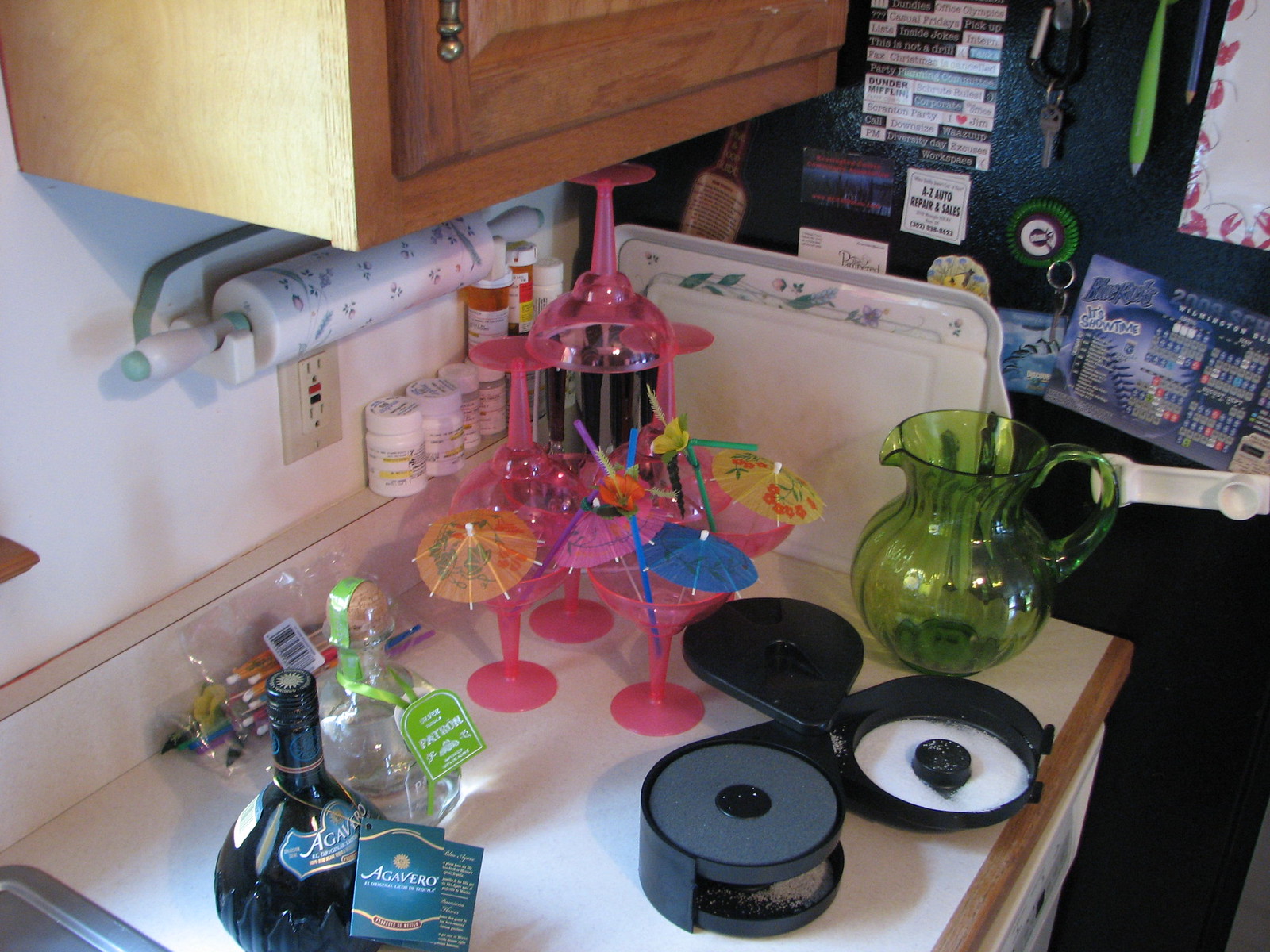This photograph captures a lively kitchen setting. In the bottom left corner, a stainless steel sink is partially visible, adding a touch of modernity. To the right of the sink, there is a collection of vibrant, vacation-themed cups reminiscent of tropical getaways like Hawaii. Each cup is adorned with colorful paper umbrellas in shades of yellow, blue, and pink, suggesting a festive, summery atmosphere. Several of the cups also contain straws in various colors—yellow, blue, and purple—indicating that they are ready for refreshing beverages. Among these, two cups are flipped upside down, standing empty.

Adjacent to the array of cups lies a large green pitcher, likely intended for serving lemonade or another chilled drink, though currently, it appears to be empty. Below this, a three-piece serving tray is stationed, with the central part being white and the flanking parts resembling disc-shaped sections. An unexplained white powder is sprinkled beneath the left disc section.

To the bottom left, a uniquely shaped bottle of alcohol marked 'Agavero' stands out. The bottle has an intriguing design, reminiscent of a light bulb or jar, adding a quirky charm to the setting. Overall, the image exudes a casual, yet festive vibe, suggesting preparations for a social gathering or a leisurely day at home.